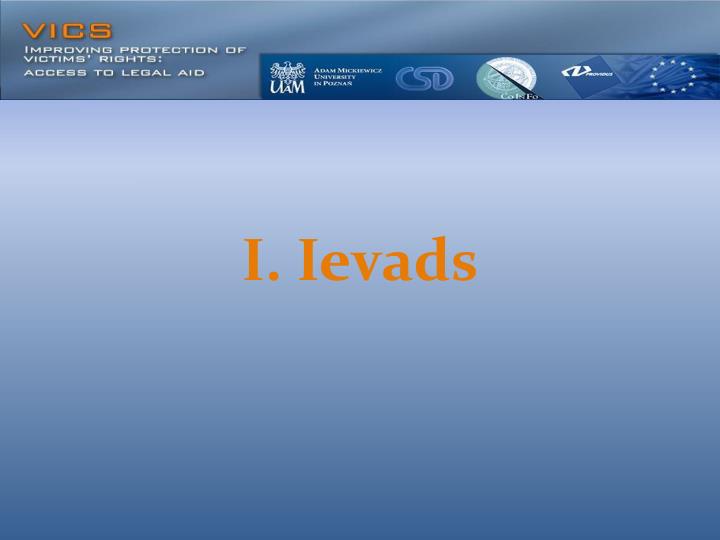The image is a detailed color screenshot in landscape orientation, combining graphic design with typography. The main color scheme is a gradient of blue and gray. At the top of the image, there is a blue and gray horizontal band featuring a visually rich wavy effect, resembling a digital fabric. On the left side of this band, written in large gold letters, is the acronym "VICS." Below this, in smaller white text, it reads, "Improving Protection of Victims' Rights, Access to Legal Aid."

To the right of this section, the band turns into a dark blue area adorned with several white insignias and fonts representing different organizations, including the logo "CSD" and "UAM Adam Mickiewicz University," indicating a connection to the University of Adam Mickiewicz in Poznań.

Beneath this primary banner, the background transitions to a lighter blue gradient, which darkens towards the bottom. Central to this area are the bold orange letters "I. IEVADS." The meticulous design and strategic use of gradients and typography emphasize the importance and formality of the content presented.